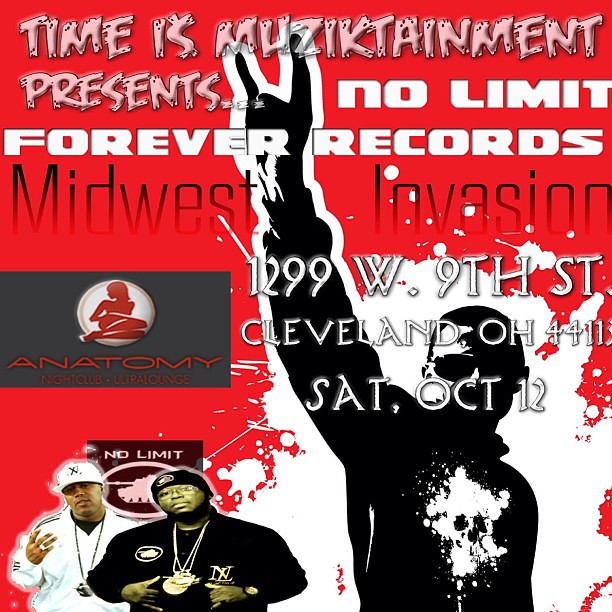The image is a vibrant digital advertisement poster for an event. It features a red background with various pieces of text in different fonts and colors. 

At the top, in pink capital letters, it reads "Time is Musictainment" with the word music creatively spelled with a 'K'. Directly below in white text, it says "Presents... No Limit Forever Records." Underneath that, "Midwest Invasion" is written prominently in black letters.

Towards the lower center of the poster, the event details are displayed in white text: "1299 West 9th Street, Cleveland, Ohio 44113, Saturday, October 12th." 

On the left side, there is a gray rectangle with "Anatomy Nightclub Ultra Lounge" written in red. Above this is a logo featuring a silhouette of a lounging woman.

In the bottom left corner, there is a photograph of two African American men who appear to be rappers. One is dressed in a white baseball cap and sweatshirt with a large pendant necklace, while the other wears a black shirt with a black knit hat and also has a large pendant necklace. Behind them, a sign reads "No Limit" along with an emblem featuring a tank.

On the right side of the poster, there is a striking black and white illustration of a man wearing sunglasses, holding up his right hand in a 'devil horns' gesture. This figure adds a dramatic flair, contrasting with the text and other images on the poster.